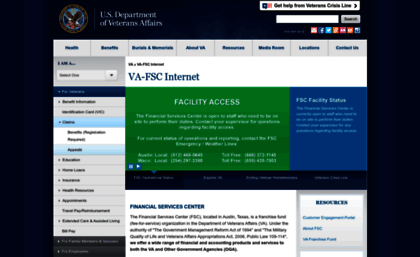Screenshot of the U.S. Department of Veteran Affairs website:

At the very top, the website features a blue header. Located on the far left of this header is a circular logo depicting a bald eagle, followed by the text "U.S. Department of Veteran Affairs." Positioned on the far right of the header is some text contained within a white box, positioned just above a search function. The search function consists of a white input box with a gray search button. Directly below these elements, social media icons are displayed.

Beneath the header, there is a navigation bar with eight different categories for users to choose from. The main body of the website is divided into a sidebar on the left and the main content on the right. The sidebar primarily features gray text with different categories and expandable dropdowns for further information.

The main content area on the right contains various sections. At the top, the text "VAFCS Internet" is displayed prominently in bold, blue font. Below this heading, there are additional sections, including a green box labeled "Facility Access" and beneath it, another label reading "FCS Facility Station." Further down are more categories to select from, followed by a white box containing a body of text. Adjacent to this, a gray box provides resource information.